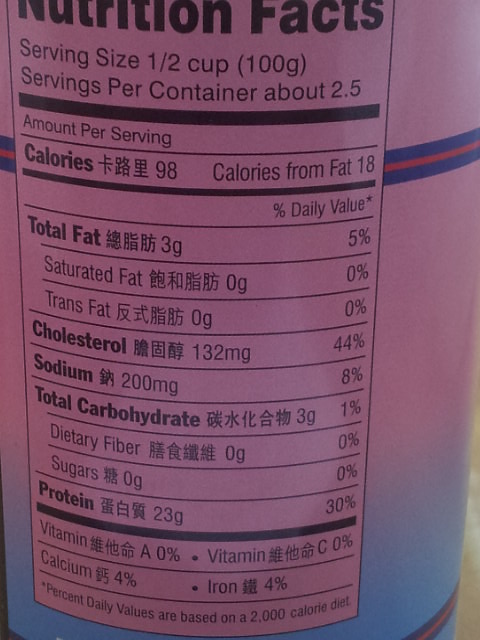The image is a close-up, portrait-oriented photograph focusing on a Nutrition Facts label affixed to a cylindrical container, likely a jar or canister. Dominating the composition is the label, which features both English and traditional Japanese text. The Nutrition Facts section at the top is distinctly pink. The upper two-thirds of the label also follow this pink theme, while the bottom portion transitions to an aqua blue through a horizontal gradient, blending like spray paint. Additionally, a navy blue stripe with a red band runs horizontally behind the Nutrition Facts area, wrapping partially around the container. The backdrop is only slightly visible, revealing a light, beach-colored surface that suggests the container is placed on a wooden table.

Detailed nutritional information includes a serving size of half a cup (100 grams), with approximately 2.5 servings per container. Each serving provides 98 calories, 18 of which are from fat. The label lists the following per serving: 3 grams of total fats, 0 grams of saturated and trans fats, 132 milligrams of cholesterol, 200 milligrams of sodium, 3 grams of total carbohydrates, 0 grams of dietary fiber, 0 grams of sugars, and 23 grams of protein. It also notes the vitamin and mineral content: Vitamin A and C at 0%, Calcium and Iron at 4%. The background information on the label highlights that the percent daily values are based on a 2,000 calorie diet. Despite these details, the exact nature of the product—whether it is a food item or a nutritional supplement—remains unidentified.